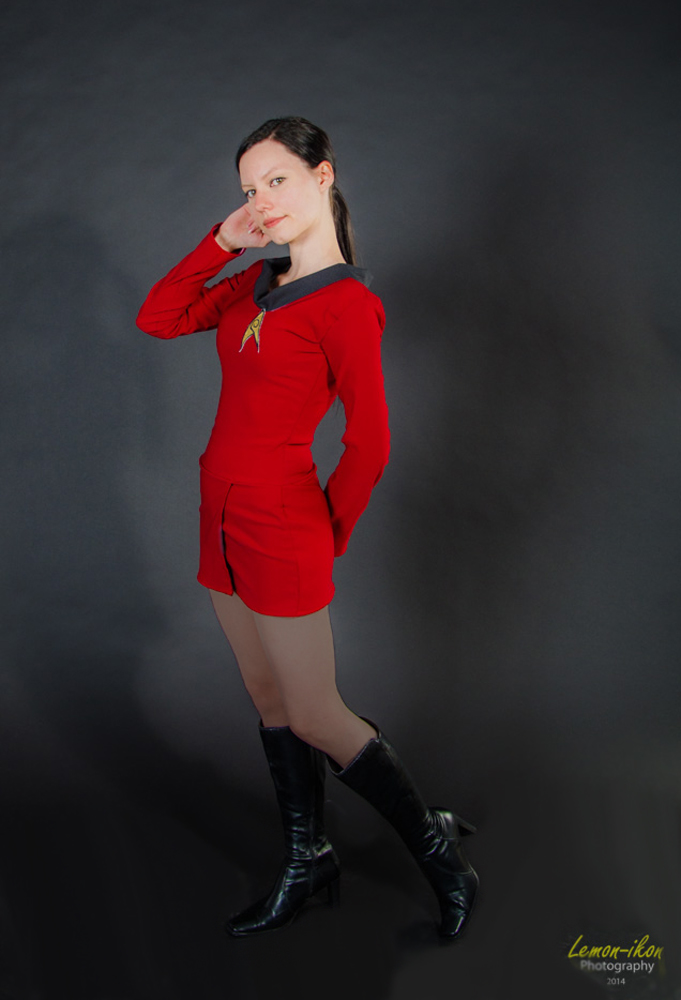The image features a young Caucasian woman, likely in her 20s, dressed in a classic Star Trek costume from the 1960s TV show. She has long dark brown hair pulled back into a ponytail, and she is striking a pose with her right hand up to her ear while her left hand is behind her back. She is looking directly at the camera. Her outfit consists of a red miniskirt dress with a distinctive yellow Star Trek Federation logo on her upper right chest, a gray collar, and long sleeves. She completes her look with shin-high black boots, evoking the appearance of a Star Trek character. The background is a dark gray abstract space, with shadows cast on either side of her. In the lower right-hand corner of the photo, the text "Lemon-Ikon Photography, 2014" can be seen.